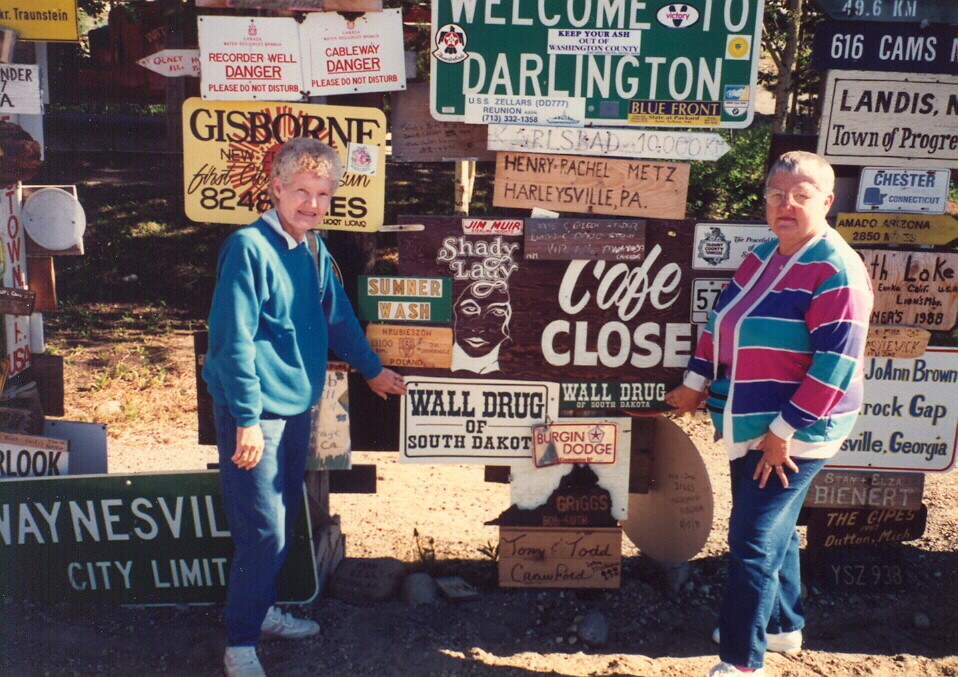The photograph captures two elderly Caucasian women standing outdoors on a sunny day, surrounded by an eclectic array of numerous signs, reminiscent of a collection one might encounter in a roadside attraction or park. The women, who appear to be in their 60s, are positioned near the center of the image, both wearing blue jeans and white pants, with the woman on the left donning a blue long-sleeved shirt with a white collar and sporting blonde permed hair. The woman on the right, with short gray hair and eyeglasses, is clad in a violet shirt topped with a multi-colored, horizontally striped jacket.

Both women are engaging with a sign that prominently reads "Wall Drug of South Dakota" and another one that states "Cafe Closed, Wall Drug of South Dakota." Various other signs fill the background, creating a vibrant and chaotic tapestry: some notable mentions include "Waynesville City Limits," "Welcome to Darlington," "Keep Your Ash Out of Washington County," "USS Sellers Reunion," "Town of Progress, Chester, Connecticut," and distances such as "10,000 kilometers" and "616 KMs." The scene is set against a backdrop of dirt, rock, gravel, and shadows with some trees whose leaves remain, suggesting cooler yet not freezing weather conditions.

The image exudes a nostalgic charm, capturing a moment of interaction and curiosity amidst a collage of historical and whimsical signs.